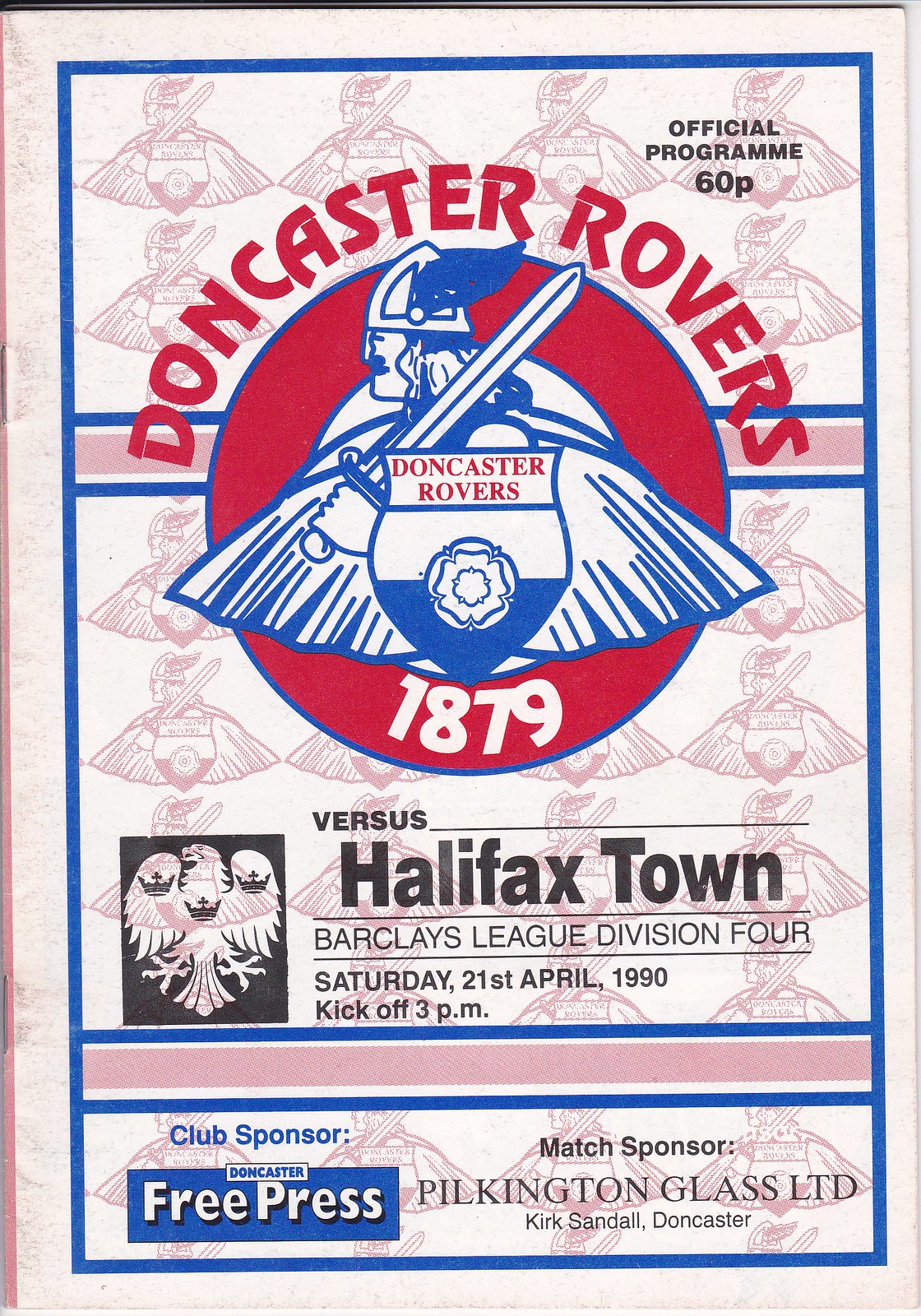This detailed image of an official soccer program for a match features prominently the Doncaster Rovers' iconic logo at its center. The logo, a Roman soldier wearing a helmet with wings, wielding a sword and donned in a cape, stands in front of a shield that reads "Doncaster Rovers" and "1879" beneath. Below the vivid red and blue emblem, the text indicates the match details: "Versus Halifax Town, Barclays League Division 4, Saturday 21st April 1990," with a kickoff time of 3 p.m. Additionally, the program highlights the club sponsor as the "Doncaster Free Press" and the match sponsor as "Pilkington Glass Ltd, Kirk Sandal, Doncaster." The image also includes a small logo with birds and intricate design elements to the side, reinforcing the historic and communal significance of the event.